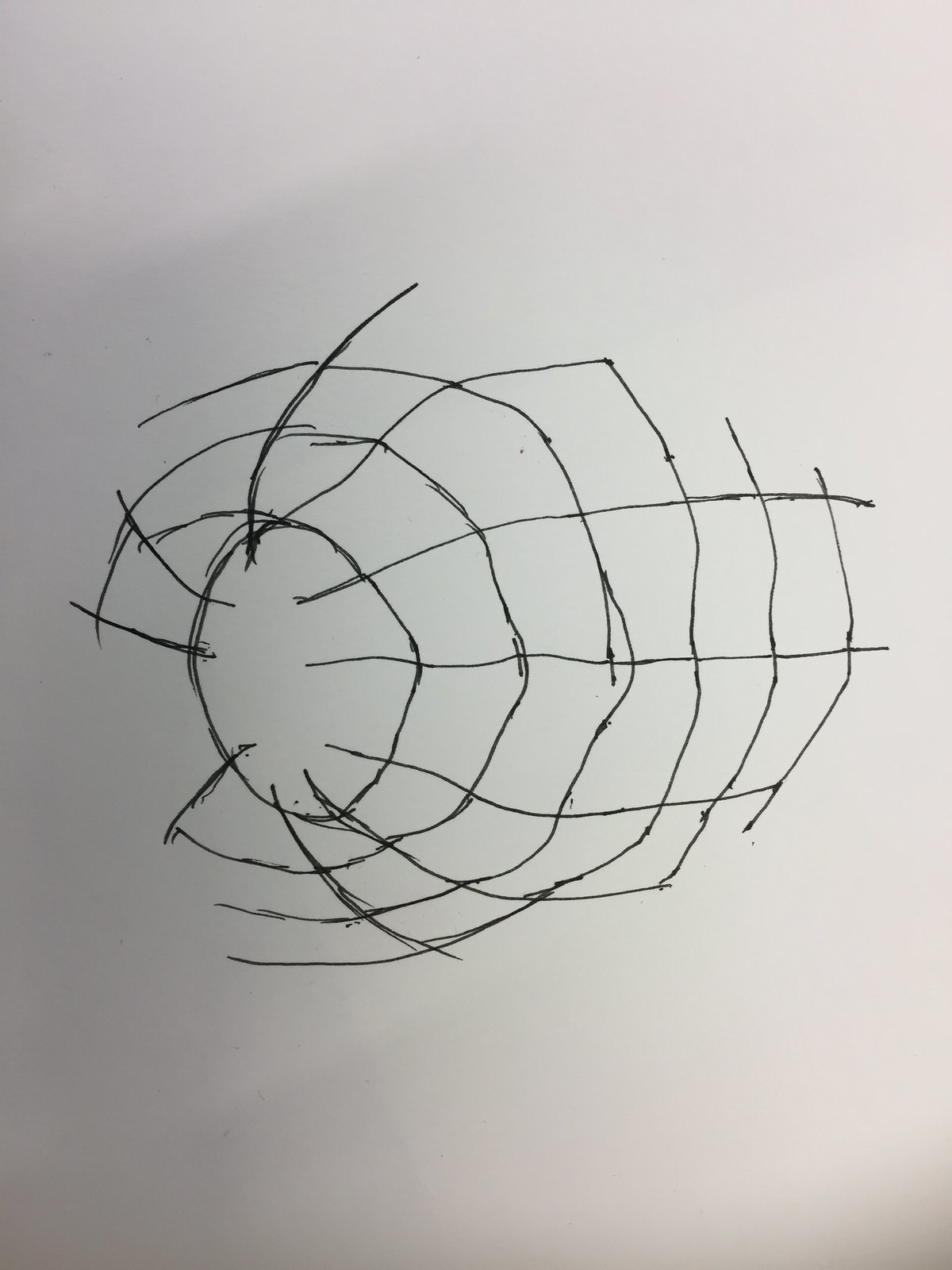A meticulously detailed pen drawing is presented on a plain white sheet of paper, open to interpretation. The illustration features a complex array of interwoven lines that might initially resemble a spider web. Upon closer inspection, the drawing appears multidimensional, evoking the form of an elongated object similar to a bullet, complete with smooth surfaces and detailed contours indicative of its shape and depth. The medium used is black pen ink, characterized by relatively thin lines. The artwork is devoid of any contextual clues or background elements, focusing solely on the intricate line work. The pattern’s design could also suggest a net-like structure or possibly even the canopy of a parachute undergoing deployment. Overall, the drawing invites viewers to explore its ambiguous yet fascinating form through varied perspectives.